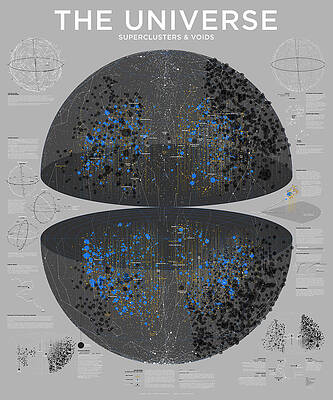This is an image of a poster depicting a 3D model of the universe. The poster has a light grey background and features prominently in the middle two dark grey semi-spheres positioned one at the top and one at the bottom, separated by a slight gap. These semi-spheres are dotted with black, blue, and yellow colors. The blue dots possibly represent superclusters, while the black areas may indicate voids. The yellow markings extend over the length of the hemispheres. At the top of the poster, white text reads "The Universe, Superclusters, and Voids." Flanking these hemispheres on the left and right sides are smaller illustrations in black and white, which resemble tiny white balls with intersecting black lines. However, the details of these smaller graphics are difficult to discern.